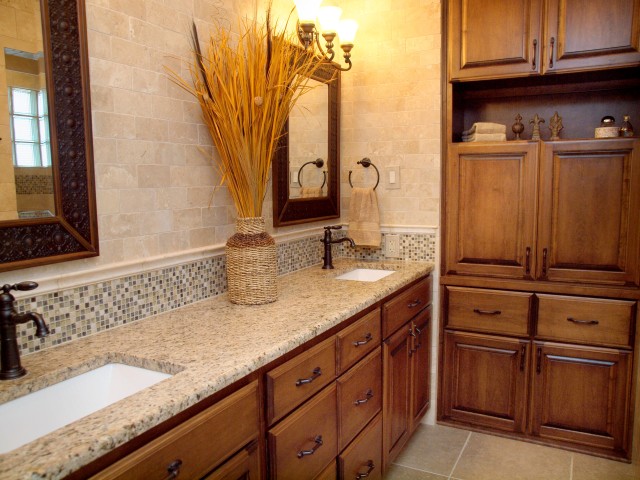The bathroom appears to be in either a luxurious home or a high-end hotel, featuring a pristine, modern design. The space is adorned with granite countertops and rich wooden drawers, cupboards, and cabinets, all of which exude a sense of elegance and sophistication. On the counter sits a decorative faux straw plant, encased in a wicker basket, with long, slender strands reaching upwards for about three feet, adding a touch of natural aesthetic.

A distinctive circular towel holder, meticulously clipped and classy, complements the polished bronze faucets, which, despite their dark hue, gleam impressively. The floor is laid with tan stone tiles, providing a warm and inviting atmosphere. The mirrors are full-size, embellished with robust, dark brown wooden frames, which lend a grounding, earthy depth to the overall decor.